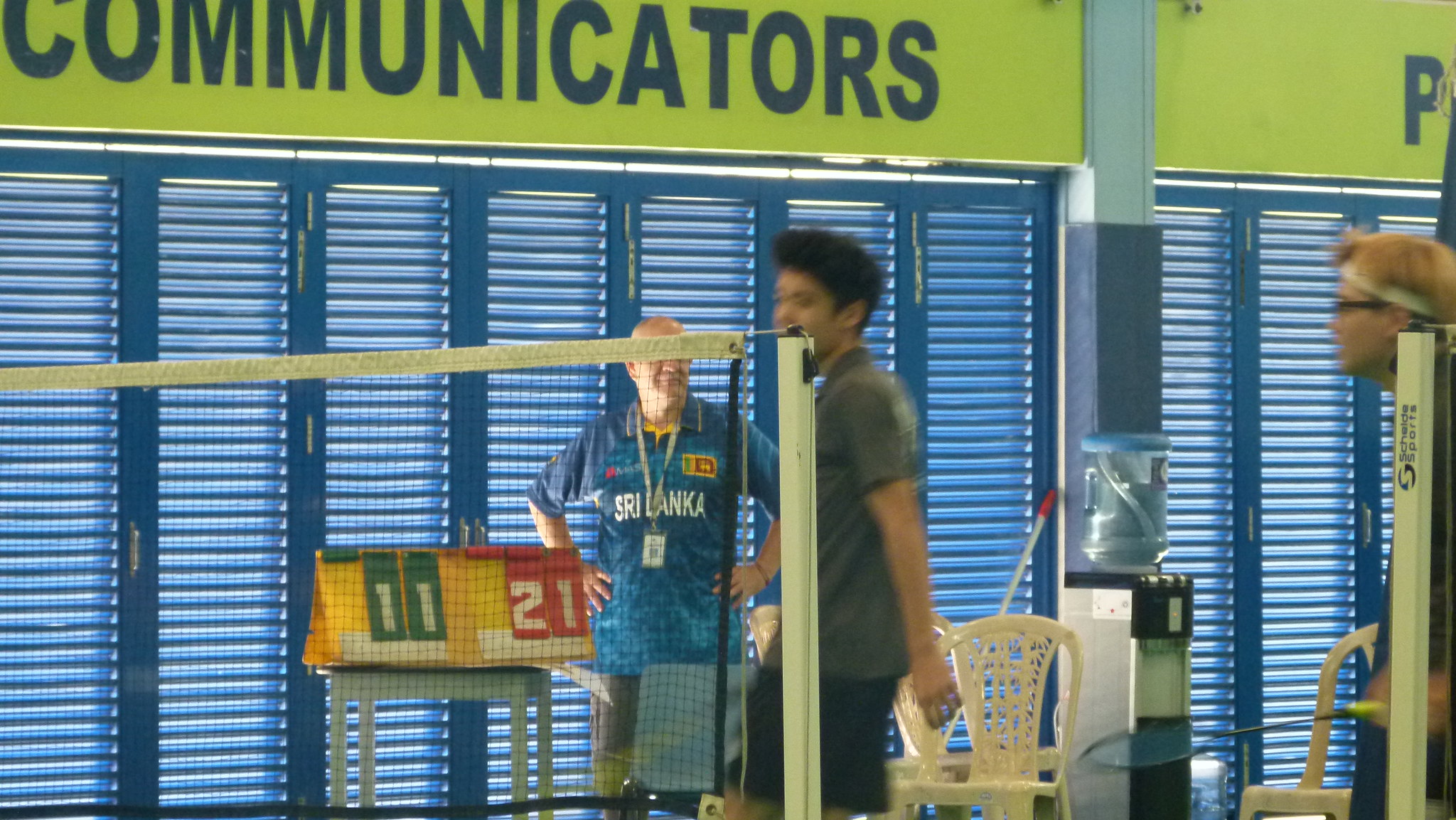The photo captures a lively scene in an indoor badminton court, situated within a building that boasts a yellow strip of wall at the top with the word "COMMUNICATORS" prominently displayed in bold, blue capital letters. The foreground features a tennis court fence, behind which three people can be seen. In the center, an older man, possibly an official, stands next to a scoreboard displaying the scores 11 (green background) and 21 (red background). He wears a blue shirt emblazoned with "Sri Lanka" in white text and gray pants. To the left, a man in a dark gray t-shirt and black shorts walks past a pole, while on the right side, a young badminton player with a headband and racket is visible, suggesting a badminton game in progress. The scene is accented with blue cabinets resembling lockers, ventilated with horizontal slats, lining the background. A white support beam stands to the right, accompanied by a water pitcher and several lawn chairs situated at the bottom-right corner, adding to the functional and organized ambiance of the gymnasium.